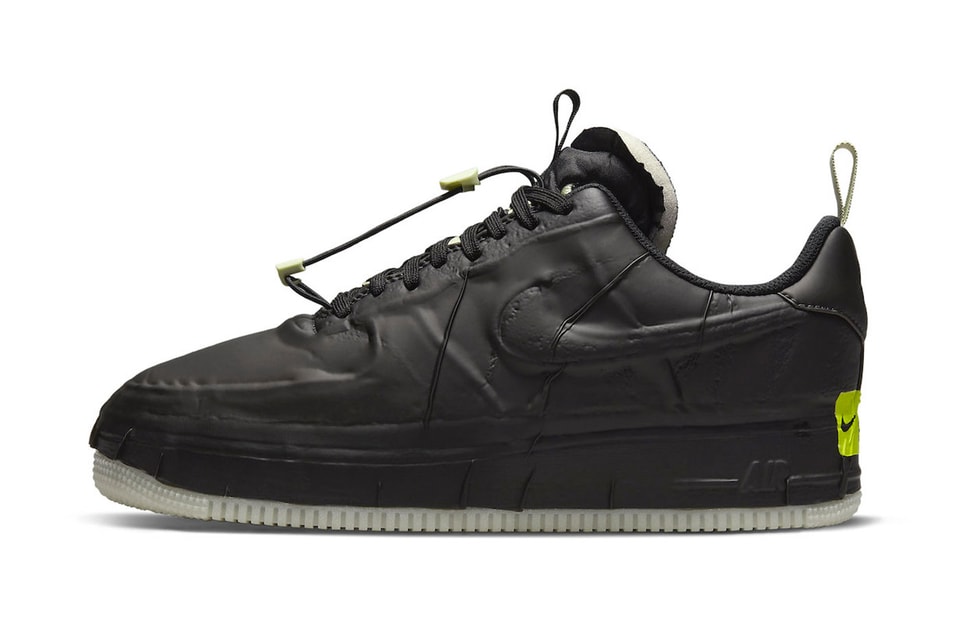In a stark white background, the image showcases a single left black tennis shoe. The upper portion of the shoe appears to be constructed from black leather, featuring intricate moldings and stitchings. This sports shoe has a prominent sole that is predominantly black on the sides, with the bottom being white and textured, waffled in appearance. The front part of the sole displays small raised dots, transitioning into ridged lines that extend from below the toes to the heel. At the very back of the heel are two rows of raised dots. A noticeable feature is a yellow rectangular or squarish shape with a black Nike swoosh embedded in the middle, extending from the back of the shoe down into the sole.

The shoe is equipped with black shoelaces, which have elastic, black stretchy connector cords with yellow connector tabs running from the top of the tongue to the bottom of the laces. The purpose of these cords is unclear. There are convenient finger pulling loops on both the tongue and just above the heel, facilitating easy wear. The tongue itself is black on the top and white on the bottom. Additionally, a white loop is present at the back of the shoe, enhancing the ease of pulling the shoe on. An edge of a green label is visible towards the sole at the back, adding a subtle detail to the overall design, which also features a black Nike swoosh molded on the side.